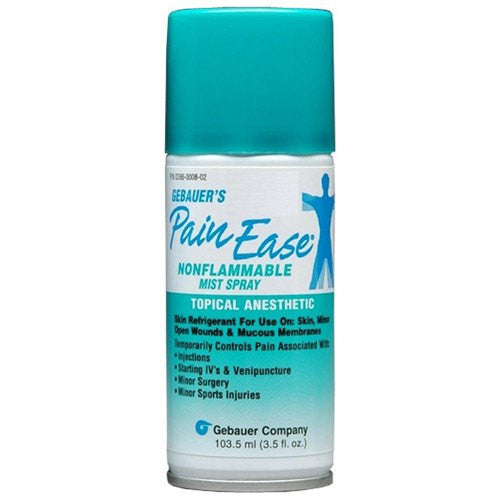The image features a cylindrical spray can of Gebauer's Pain Ease, a non-flammable mist spray designed for topical pain relief. The can is primarily aqua blue with a matching pull-off cap, accented with sections of white and green. The top section with a white background displays the brand name, "Gebauer's" in blue text, followed by "Pain Ease" and "Non-Flammable Mist Spray" in black and green print, respectively. An outline of a person shaded in blue is also present on this section. The midsection against a green background states "Topical Anesthetic" in white capital letters, and additional information in black text explains it is a "Skin Refrigerant for Use on Skin, Minor Open Wounds, and Mucous Membranes," useful for "temporarily controlling pain associated with infections, starting IVs and venipuncture, minor surgery, and minor sports injuries." The bottom part has the company logo in blue, the name "Gebauer Company," and indicates the can contains "103.5 milliliters (3.5 fluid ounces)." The overall color scheme of the can is predominantly aqua blue, white, and black.